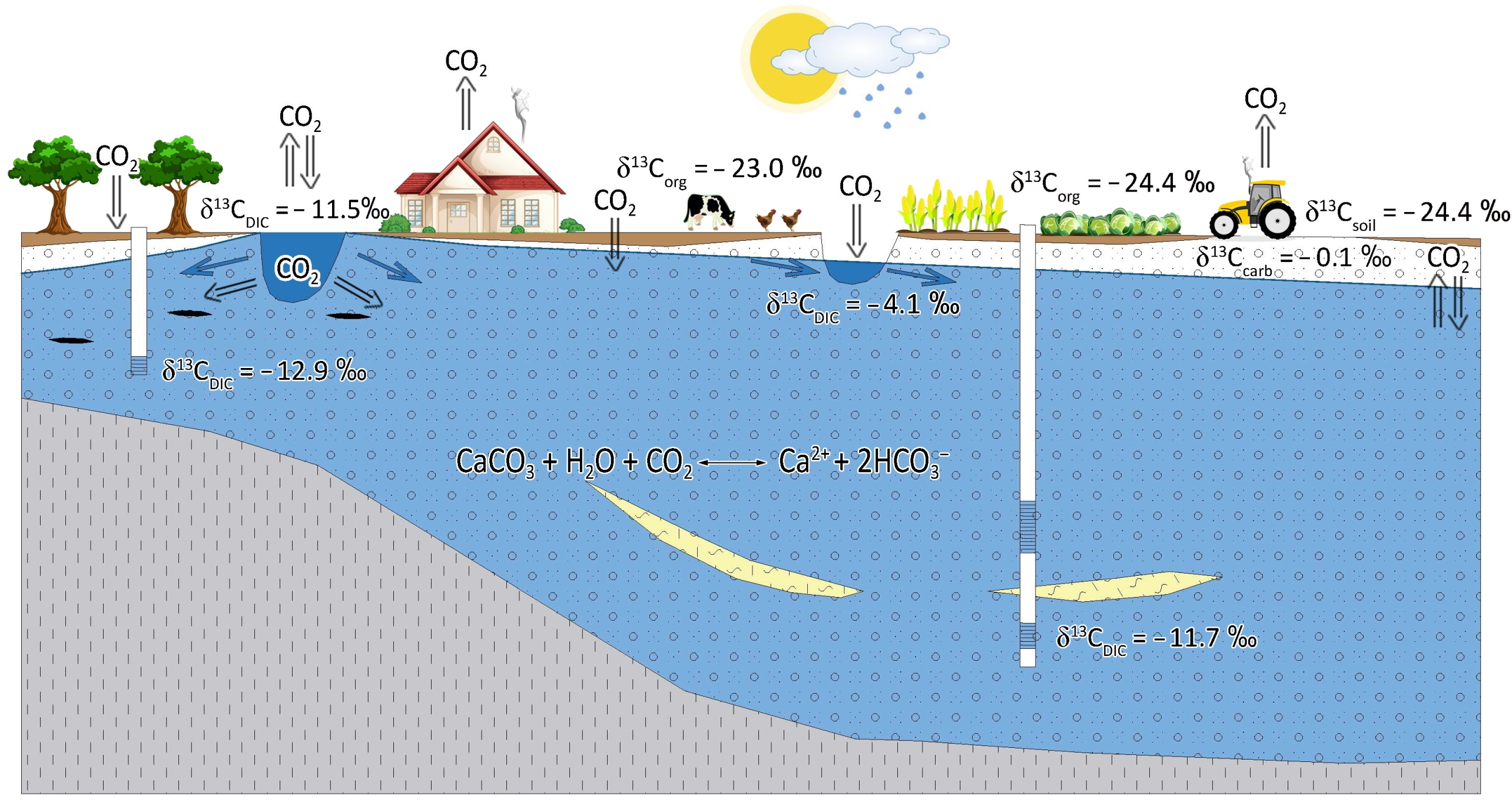The image, rendered in a cartoon style against a white background, intricately illustrates the carbon dioxide (CO2) cycle and its interactions with various natural and human-made elements. Against a clear, white sky featuring a radiant sun and scattered clouds releasing droplets of precipitation, a diverse landscape unfolds. On the left, tall, green trees are depicted absorbing CO2, which is shown seeping into a water source beneath them—complete with complex, if not perplexing, mathematical formulas and chemical equations indicating the mechanisms of CO2 absorption. To the right, a cozy house releases CO2 into the atmosphere, followed by a scene of farm animals, including cows and chickens, contributing to CO2 emissions. Further to the right, flourishing cornfields and other vegetables like lettuce are shown, accompanied by a tractor emitting CO2. Throughout the image, arrows demonstrate the movement and transformation of CO2, depicting its journey through the environment. Despite the absence of a title, the graphic uses detailed computer-generated visuals to convey the intricate dynamics of CO2 release and absorption in an ecosystem, offering a comprehensive view of this vital environmental process.